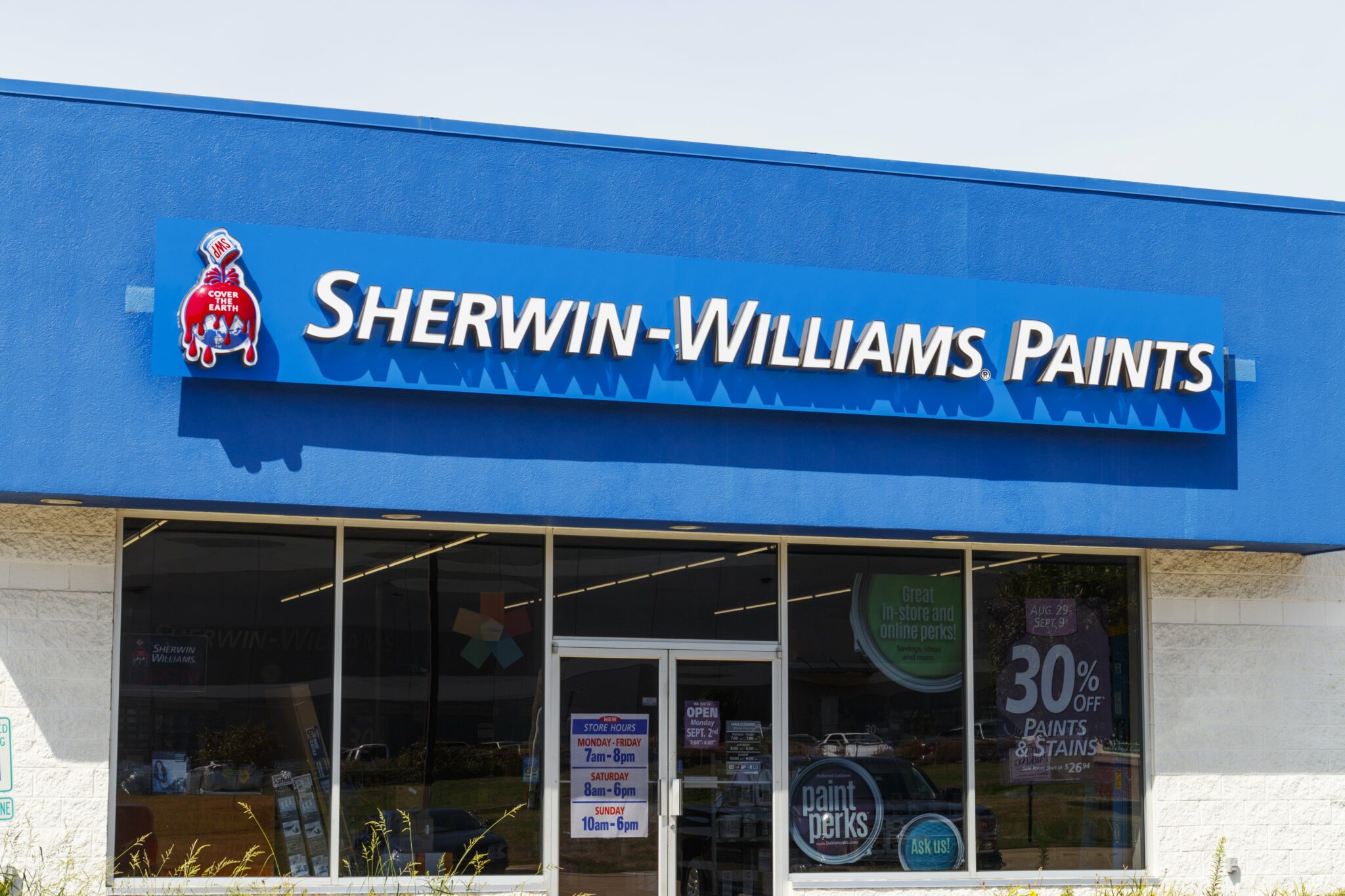This outdoor photograph captures a bright, sunny day with a clear, pale blue sky devoid of clouds. Dominating the scene is a storefront featuring a striking blue roof and a matching blue sign with white lettering that reads "Sherwin-Williams Period Paints." To the right of the store name, there's a small light blue square, and to the left, a graphic illustration of a can spilling red paint. 

Below the sign, the store entrance is comprised of four large glass panes and double glass doors that invite customers inside. The storefront is adorned with planters filled with ornamental grasses situated in front of the windows. The windows display promotional signage announcing "30% off paints and stains" and highlighting "Paint Perks." Additional signs on the glass doors provide operating hours, though they are too small to decipher in the photograph. The bright sunlight casts a distinct shadow beneath the signage, and the interior lighting of the store, mainly track lighting on the ceiling, is faintly visible through the glass.